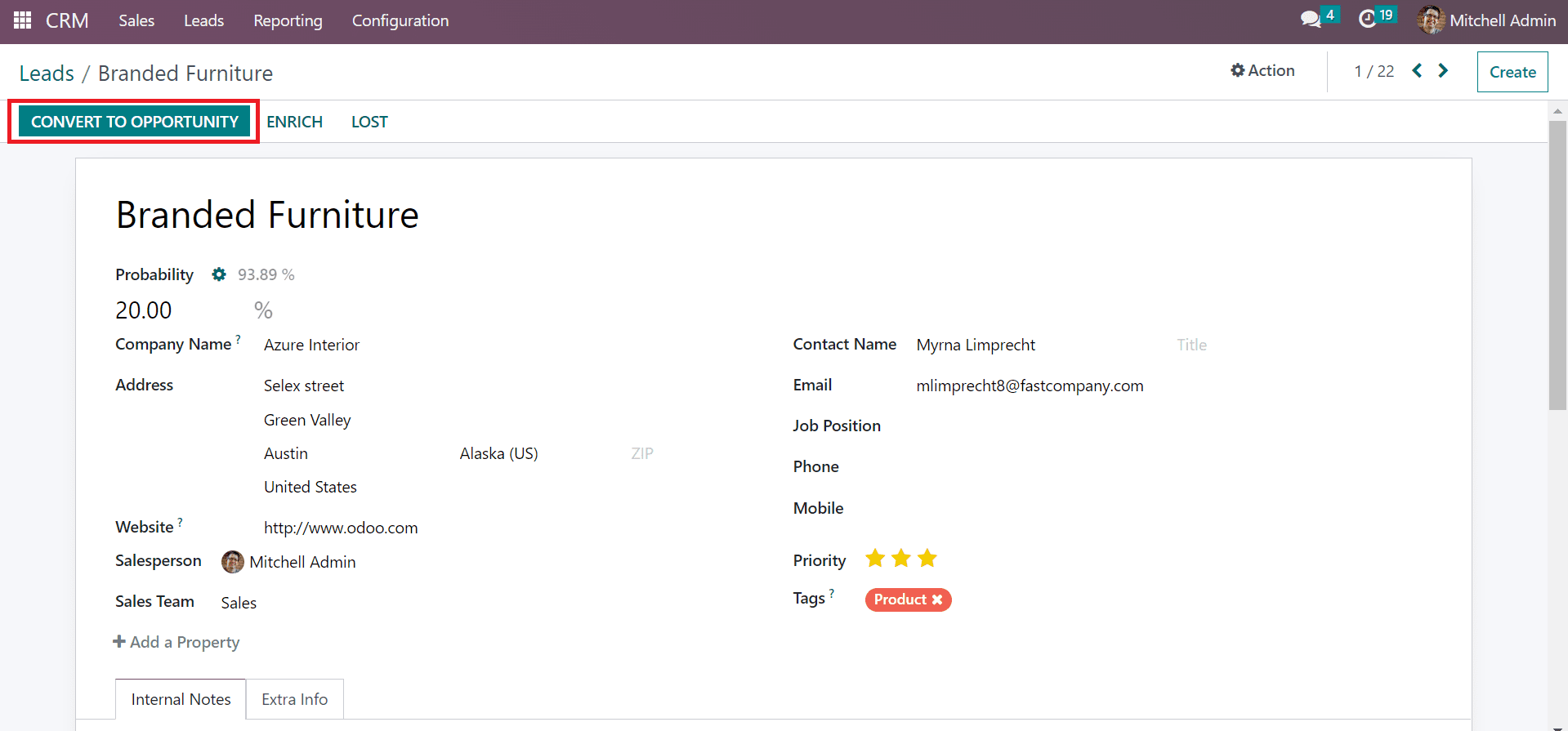**Descriptive Caption:**

The website features a prominent burgundy banner at the top with a white square comprised of nine smaller white squares. To the right of this white square, there are the white uppercase letters "CRM". Beside this label, four white tabs are aligned, labeled "Sales," "Lease," "Reporting," and "Configuration." Directly below this banner, the text "Lease/Branded Furniture" is clearly displayed.

Immediately beneath this section, there is a small red rectangle outlined in red, containing a green rectangle with the white text "Convert to Opportunity." Next to this, in green letters, are two tabs labeled "Enriched" and "Lost." 

Below these tabs is the text "Branded Furniture." On the left side, detailed information is presented as follows:
- Probability: 93.89%
- Probability: 20.00%
- Company Name: Azure Interior
- Address: Southern Street, Green Valley, Austin, Alaska, United States
- Website: http://www.odoo.com
- Salesperson: Mitchell Admin
- Sales Team: Sales

On the right side, more contact details are displayed:
- Contact Name: Myrna Limprecht
- Email: M-L-I-M-P-R-E-C-H-T8@fastcompany.com
- Job Position, Phone, Mobile
- Priority: Three yellow stars
- Tag